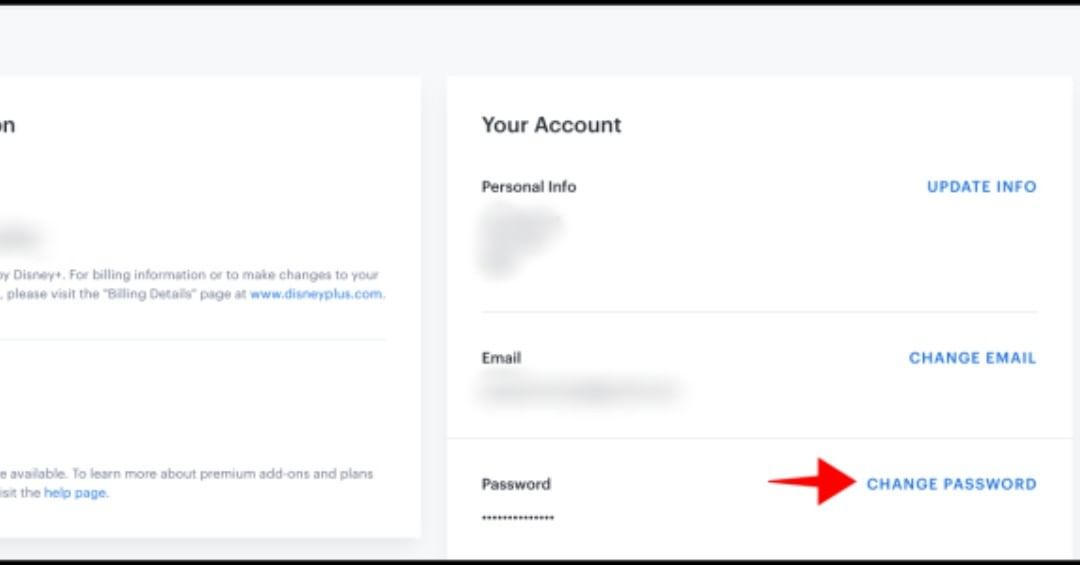This image is a screenshot of the account settings page for Disney Plus, specifically focusing on the billing information and personal details section. The layout is horizontally oriented, with thin black borders at the top and bottom of the image. The upper portion of the screen features a light bluish section that transitions to white as it moves across from left to right and then back under to the left.

On the top left, there is a black letter "N" indicating navigation options, accompanied by smaller text confirming that this is indeed a page related to Disney Plus billing information, along with the website address. The footer of the image contains additional black text on add-ons available for the service.

Towards the right of the image, a clearly defined white square occupies the page, bordered lightly by a thin blue line. The upper left corner of this square contains the label "Your Account" in black, followed by "Personal Information," with the relevant personal details blurred for privacy. Adjacent to these sections, there's an "Update Info" option in blue text.

Beneath this, the "Email" section displays the user's email, also blurred out, with a "Change Email" option in blue to its right. Following this, the "Password" section features obscured password characters represented by dots, with a "Change Password" option in blue positioned to the right. Notably, a prominent red arrow points to the "Change Password" text, drawing particular attention to this option.